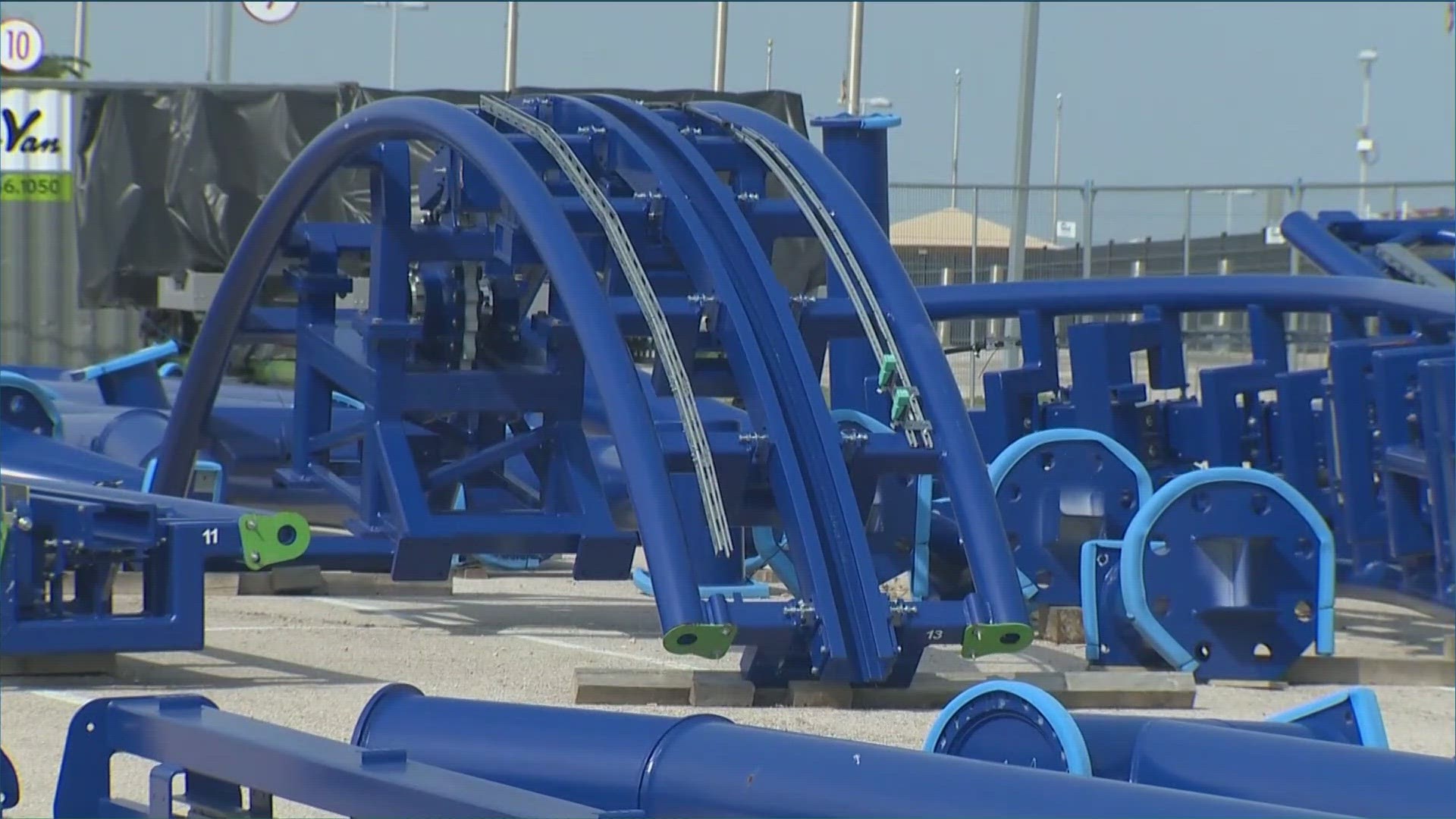This detailed photograph, captured in landscape orientation, showcases an outdoor construction area filled with large, metallic structures uniformly painted in bright blue. Central to the image is a notable semi-circular or arc-shaped structure with multiple cross pieces, resting side by side and open underneath. The scene is characterized by a concrete surface where the blue metallic components are arranged somewhat randomly, each with visible bolting points. On the right side, there are several wheel disc-shaped objects with blue styrofoam around their edges. Additionally, there are angled, curved pieces possibly hinting at components for carnival equipment. A gray chain-link fence lines the background on the right, alongside a grey-colored metallic wall, while a tin container covered by a black tarp is visible on the left. Tall steel poles, some possibly with lights, rise behind the chain-link fence. The photograph is set against a light blue sky, presenting a vivid contrast to the industrial scene below.